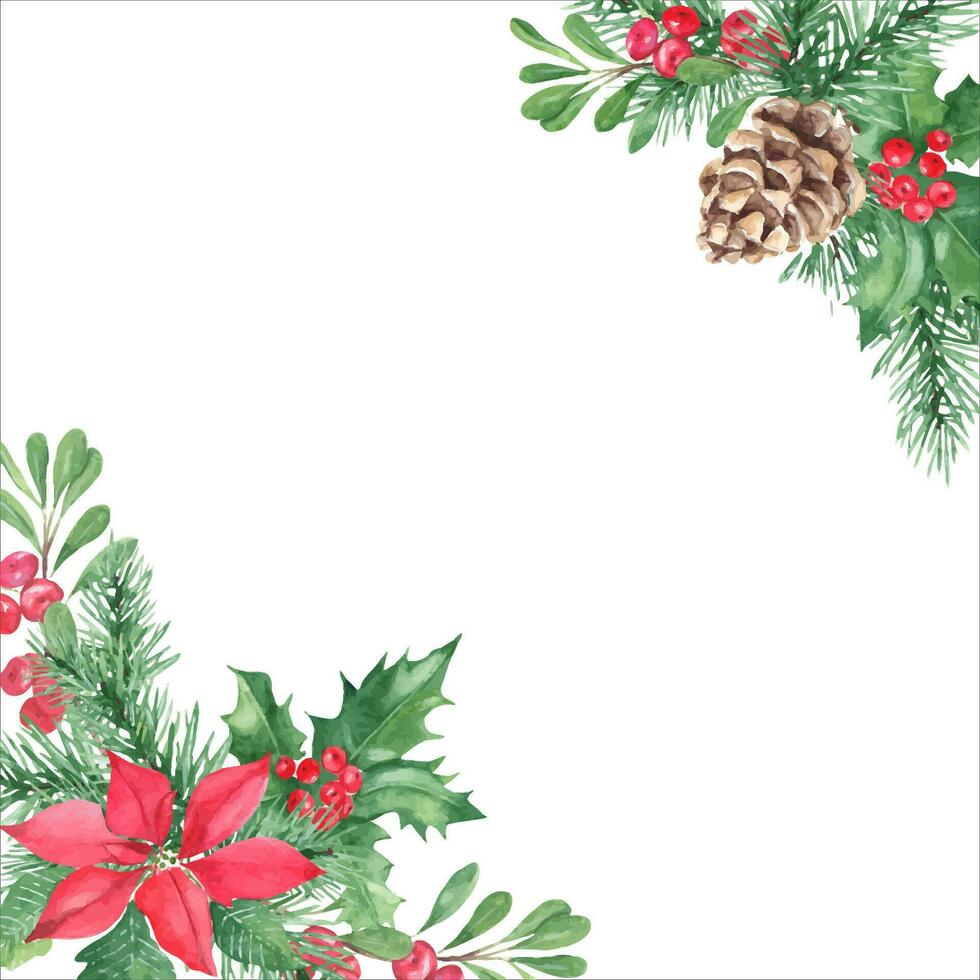This image depicts a piece of white stationery, adorned with festive graphics that lend a Christmassy feel. Positioned in the bottom left corner is a red poinsettia, surrounded by an assortment of green leaves and pine needles, with small round red berries interspersed. The berries and pine needles display hints of white, suggesting a touch of frost. In the top right corner, there is a cluster of green leaves of various shapes encircling a large brown pine cone, which also has subtle accents of white. Together, these decorative elements frame the otherwise blank and white page, creating a seasonal and festive atmosphere.